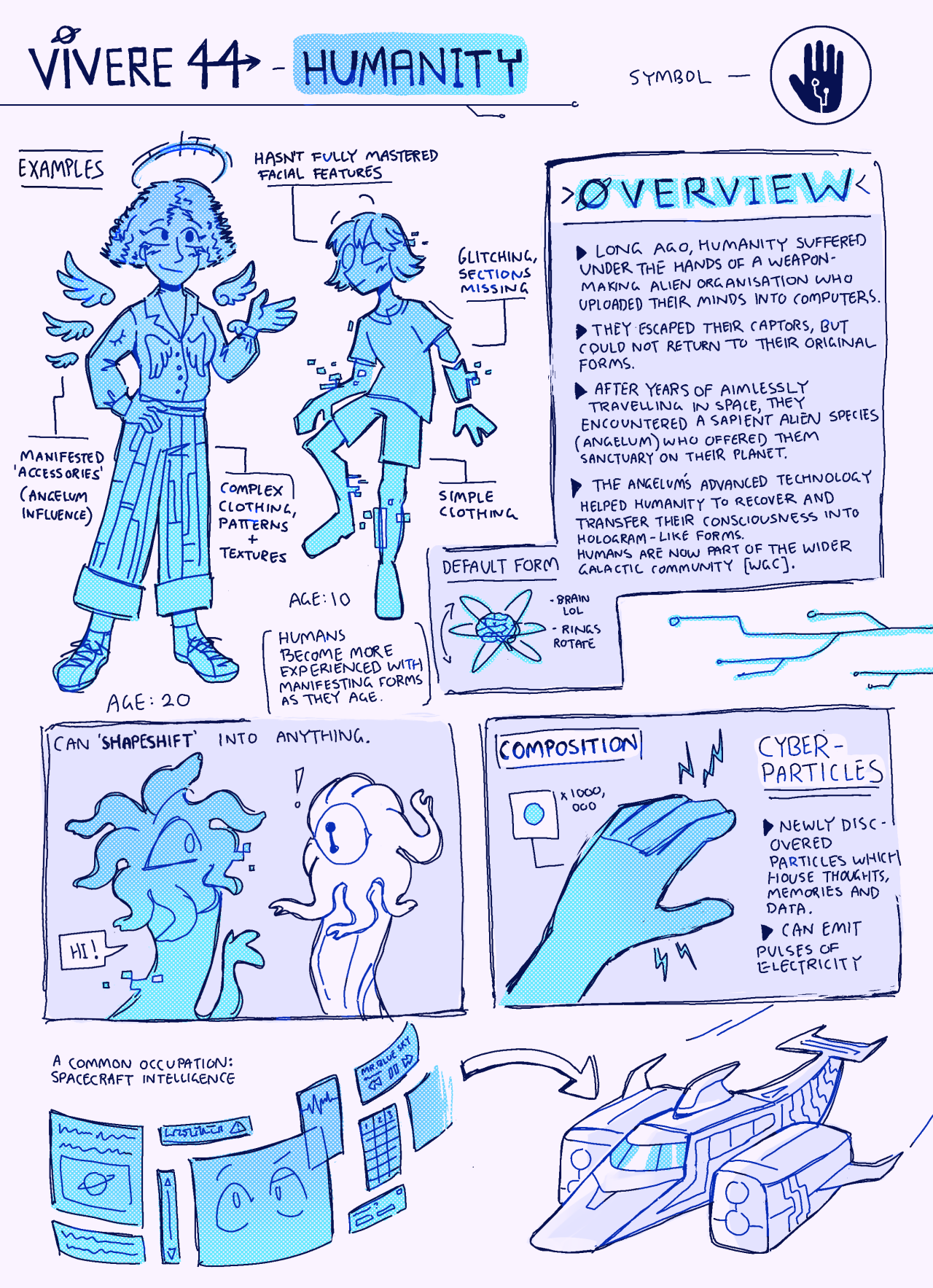The image is an intricate drawing resembling a comic strip titled "Vivere 44 Humanity." At the very top, it features a small drawing of planet Saturn and the word "VIVERE" in bold letters, followed by the number 44 and the text "slash humanity." To the top right, there's a black palm print with the word "overview" beneath it, detailing four key points. The story begins with humanity suffering under the control of a weapon-making alien organization that uploaded human minds into computers. Eventually, humanity escapes but cannot return to their original forms. After years of aimless space travel, they encounter an advanced sapient species called Angelum, who offers them sanctuary, allowing them to transfer their consciousness into hologram-like forms using sophisticated technology.

The illustration includes two central humanoid figures in the upper left. One appears to be a winged woman with complex clothing patterns, indicating a higher level of manifested accessories and an age of 20. The other figure is a smaller, blue character, seemingly young and glitching, reflecting their simpler clothing and age of 10. Text around these figures explains that humans become more skilled at manifesting their forms as they age.

On the right, there's a depiction of two shape-shifting creatures exchanging greetings, alongside a blue hand and arm emitting electric pulses, symbolizing newly discovered cyber particles that house thoughts, memories, and data. Additionally, panels show a spaceship connected to a series of diagrams illustrating spacecraft intelligence, a common occupation in this new galactic community. The complexity of the details, from the symbolic logos to the narrative captions, weaves a vivid story of humanity's adaptation and integration into a wider galactic society.